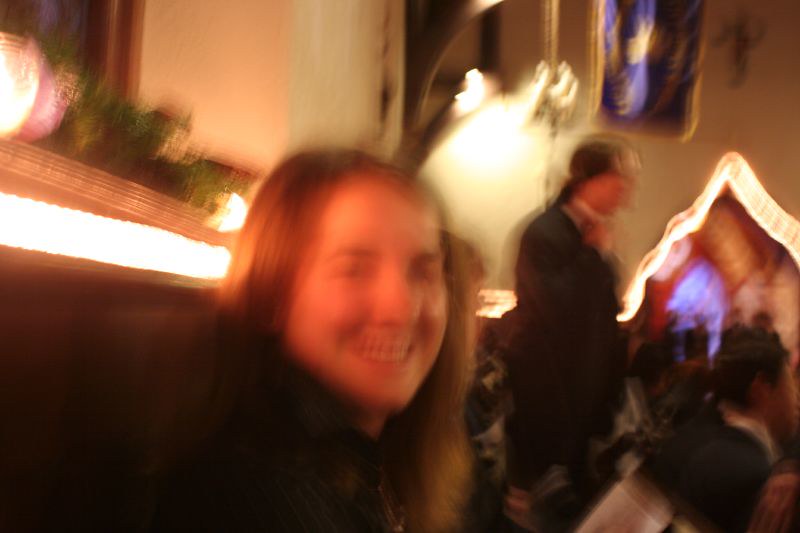In this blurry, out-of-focus indoor scene, a woman with long brown hair, dressed in a black shirt with white lines, sits on a brown bench situated towards the center-left of the image. She is smiling warmly and looking directly into the camera. Behind her stands a man with longish brown hair, clad in a brown coat. In the background, several people, indistinct due to the image's blur, move through an illuminated archway on the right. The wall behind them is white, adorned with colorful flags, including a purple and gold one in the upper right, as well as a blue and silver blanket hanging down. The setting, possibly a church or a similar venue, includes a mantelpiece or a light that spans from left to right behind the woman's head, enhancing the ambient indoor scene.